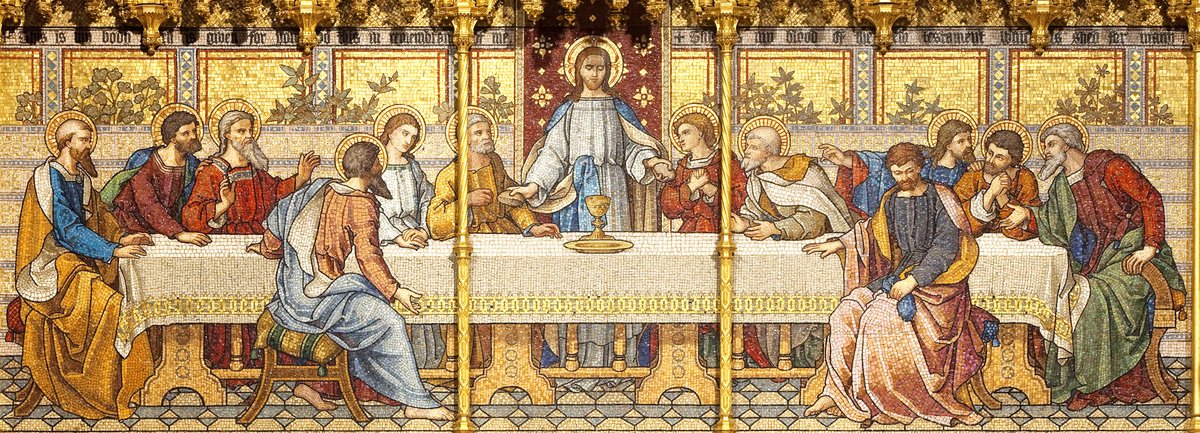In the image, a vivid and detailed portrayal of the Last Supper is displayed, crafted by an artist whose style diverges from the realism of Leonardo da Vinci’s more famous work. The scene captures Jesus Christ standing at the center of a very wide table adorned with a white tablecloth featuring a gold trim. Jesus, depicted with a halo behind his head, gazes down at a golden chalice before him, embodying the moment of communion. Surrounding him are his disciples, each with halos except for Judas, who is on the opposite side with his back turned, devoid of a halo, and seemingly disengaged from the central event.

The painting is rendered in rich colors, including shades of orange, white, blue, green, red, yellow, and pink, providing a vibrant and lively atmosphere. The disciples, draped in flowing robes of various colors, are mostly seated along the far side of the table, with two figures on the near side, one on the left and one on the right. The overall scene is set against a background infused with natural lighting, highlighting the clarity and detailed textures of the image. The floor features an intricate blue and cream-colored pattern, complementing the decorative panels and vines that adorn the back wall. Additionally, there appears to be some text inscribed at the top of the image, presumably echoing the words of Christ during the Last Supper, enhancing the narrative depth of this artwork.